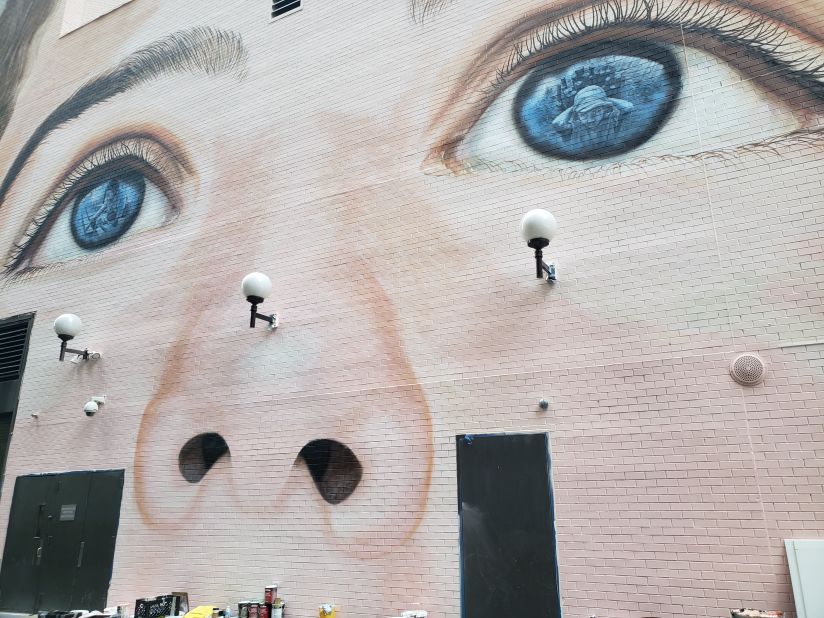The image depicts a large-scale mural adorning the brick side of a building, captured from a street-view perspective. The artwork is a close-up of a person's face, spanning approximately 50 feet in height. Dominated by deep set blue eyes, the mural features intricate details within the pupils. In the right eye, the reflection shows a young boy, seemingly holding sticks and wearing a hat, with a city skyline in the background. The left eye reveals another figure, possibly a woman, reaching out towards something. The mural is situated above two black doors and is flanked by three white lamps, with several paint cans visible at the base, suggesting recent completion. The artwork is a striking example of urban street art, blending vivid imagery with a powerful use of color and perspective.